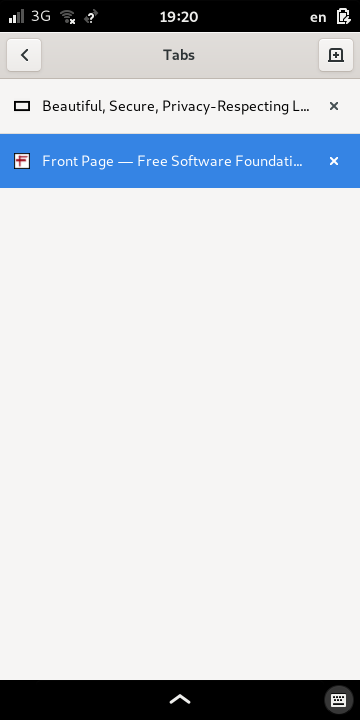This image is a screenshot from a smartphone displaying a web browser interface. At the very top, there is a status bar on a black background that includes a 3G phone service indicator, a question mark beside an inactive Wi-Fi icon, the time displayed as 19:20, an "EN" language indicator, and a battery charge icon.

Beneath this status bar, there is another strip featuring navigation elements. On the left, there is an arrow icon, while the center displays a "Tabs" header in gray. To the right, there is a box with a plus sign, indicating the option to open a new tab.

Below this navigation strip, the screenshot shows two browser tabs. The first tab, labeled "Beautiful Secure Privacy Respecting," has an "X" icon next to it for closing the tab. The second tab, highlighted in blue, reads "Front Page - Free Software Foundation" and also has an "X" icon for closing it.

The main content area below these tabs is largely empty, filled with an off-white background. At the very bottom of the image, there is a black bar containing an upward arrow, presumably to open additional options or close the current view.